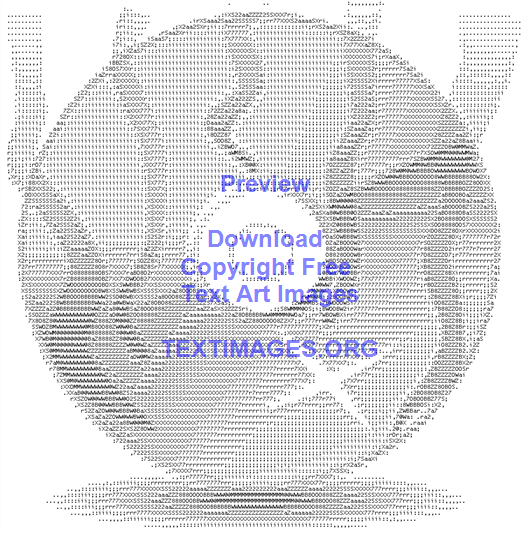This image showcases a central design, resembling a spherical or circular object, set against an all-white background. The design, which may evoke the appearance of a billiard ball, golf ball, or even a CD from the 80s or 90s, is intricately crafted with myriad tiny black and white text elements, possibly including X's, Y's, numbers, dots, and commas. Positioned precisely at the center of the image, the circular artwork casts a subtle shadow on the ground, enhancing its three-dimensional effect. The perimeter of the circle features numbers in succession, and inside the circle, there are dark gray, worm-like squiggly lines that extend outward. Overlaying the design is a light purple text reading "Preview. Download copyright-free text art images textimages.org," serving as a watermark. The image reflects a sophisticated piece of digital text art, possibly mimicking the output of an old dot matrix printer.